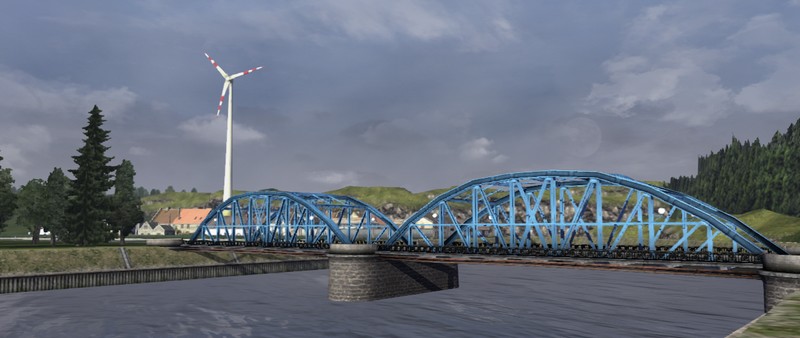This is a wide, horizontally aligned rectangular image, showcasing a detailed outdoor scene centered around a striking blue bridge with two distinctive arches on each side. The sturdy support structure of the bridge appears to be composed of gray brick and concrete, indicating a traditional yet robust design. Below the bridge spans a body of water, reflecting a dark grayish-blue hue, contributing to the overall serene yet somber atmosphere of the image. 

To the left of the bridge, there stands a tall, white wind turbine with three prongs marked by red stripes, indicative of renewable energy technology. The scene further features varied tree life: a prominent tall tree surrounded by shorter trees on the left, and an expansive section of dark green wooded area on the right. Just behind the bridge on the right side, one can observe rolling hills covered with grass and a dense assembly of evergreen trees.

The sky overhead is a blend of gray and feathery light gray clouds, evoking a dreary, overcast day. This atmospheric backdrop subtly enhances the natural and structural elements of the scene, meshing the modernity of the bridge and wind turbine with the timelessness of the natural landscape. Some minor hills in the background add depth and dimension to this expansive view, making the image feel panoramic and immersive.